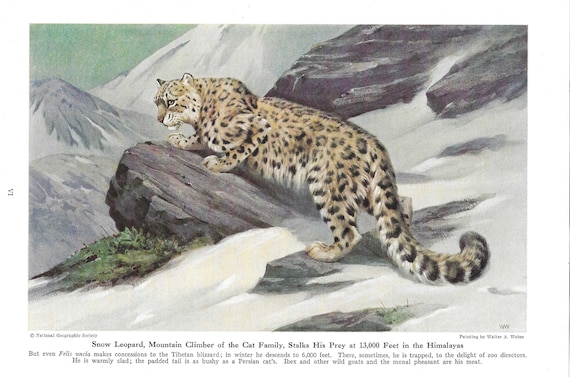This watercolor painting, possibly featured in a nature magazine or book, showcases a majestic snow leopard perched on a rocky cliff amidst a snowy landscape. The detailed illustration, set against a soft blue sky with snow-covered mountains in the background, captures the snow leopard in a moment of poised alertness as it appears to be stalking its prey. The scene includes a patch of green grass beneath a prominent boulder, with the snow leopard’s tan, black, and white fur standing out vividly. Its two front paws are placed on the rock, as if surveying the surroundings, with its head positioned in the upper left and its tail in the lower right. Beneath this captivating image, black text reads, "Snow Leopard: Mountain climber of the cat family stalks his prey at 13,000 feet in the Himalayas." Additional smaller text is present but too tiny to decipher. The overall imagery and layout give off a slightly vintage feel, adding to the timeless nature of this powerful big cat.